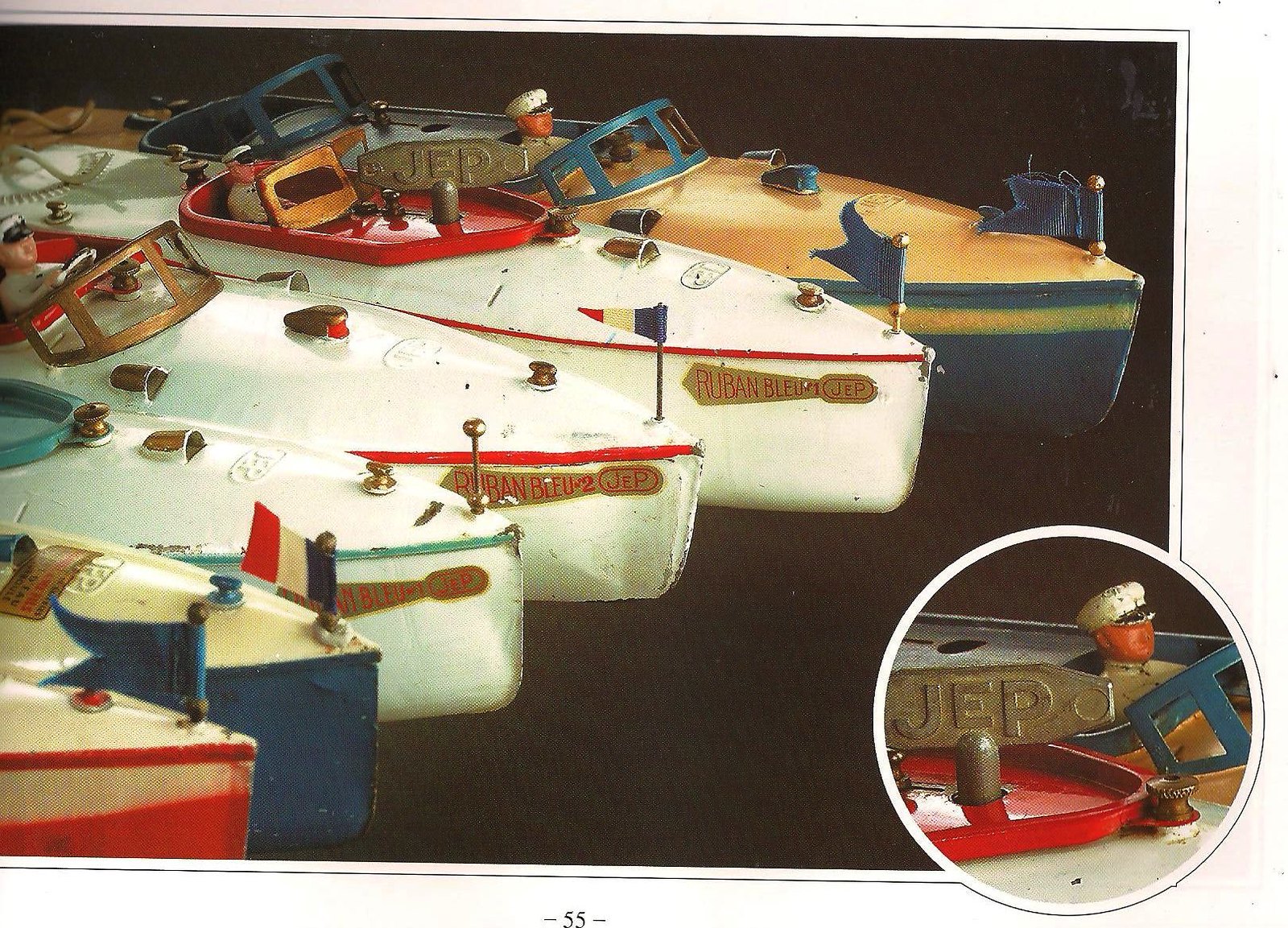This photograph features a collection of six vintage toy speedboats, arranged diagonally from the bottom left corner to the upper right. The boats, which appear to be made of wood, are displayed against a dark, brownish-black background, giving a dramatic contrast to their colorful exteriors. Each boat is distinctively painted in vibrant colors—white, red, blue, green, and yellow—and most of them carry small flags at their fronts, though one lacks a flag. These boats display details characteristic of old-fashioned speedboats, including short windshields and a streamlined design.

A notable feature in the bottom right corner of the image is a circular close-up showcasing the last boat, a yellow and blue vessel. Inside this zoomed-in detail, there’s a small figurine of a sailor wearing a white cap and suit. This boat also prominently features a metal casting labeled "JEP," which seems to be a common mark, as it appears on the fronts of most of the boats, including one with the name "Ruben Bluem."

The boats are positioned from the largest to the smallest along the scene. The largest boat, tan with green trim, dominates the foreground, followed by a progression of smaller boats, including white vessels with varying trims. Despite their miniature scale, the intricate details, such as the presence of drivers in some, emphasize the craftsmanship of these toys.